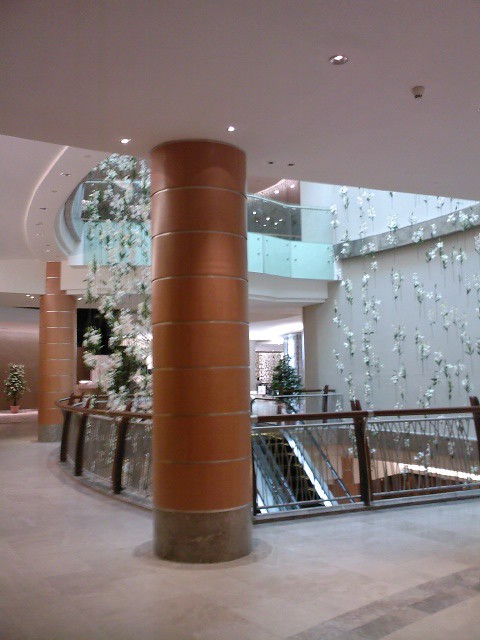The image depicts an indoor scene of a splendidly decorated building, likely a shopping mall or convention center, seen from an intermediate level—the second of three visible floors. Central to the photograph is an asymmetrical multi-level opening, edged by a sophisticated mix of brass or bronze-colored concrete and metal support beams with gray accents. In the background, an escalator ascends from the first to the second floor, flanked by elegant glass railings supported by wooden handrails and poles on both the current and upper levels.

The floor the photographer stands upon is a subtle gray or tan shade, possibly featuring a square-carpeted pattern. Overhead, the white or light gray ceiling, which forms the base of the third floor, is adorned with oblong silver hanging decorations, likely flowers, suspended from strands originating above. These festive elements, including Christmas trees on the lower left and in the right center of the picture, contribute to the elaborate décor.

The photograph captures additional details such as plants, doorways, and ceiling lights on the second and third floors, enhancing the visual richness. Notably, another brass and silver support pillar, visible on the far left, upholds the third floor. The overall ambiance suggests a well-decorated interior designed for a significant commercial or public space, with decorations contributing to a seasonal festive atmosphere.